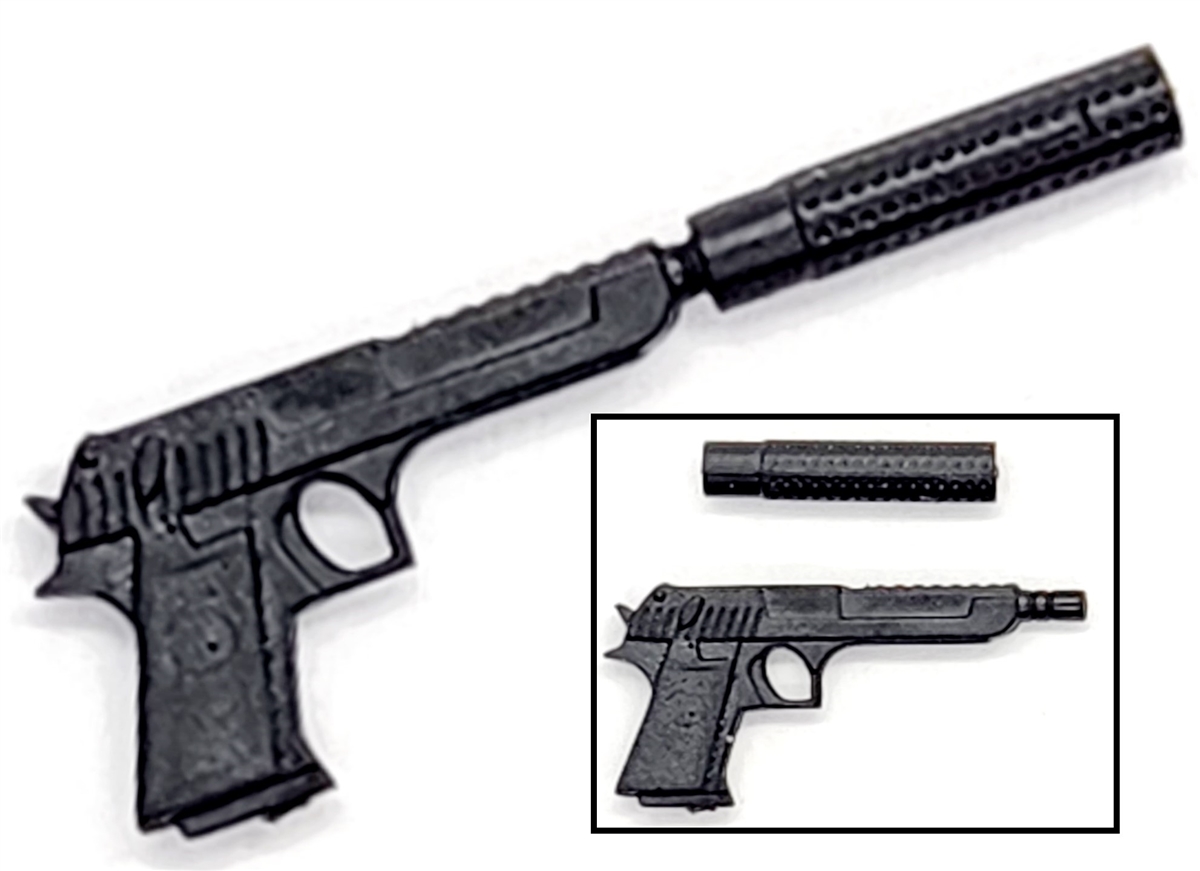The image depicts a low-resolution photograph of a peculiar black gun with an attached silencer, positioned against a white background. The gun's design appears unconventional, lacking a visible trigger, which raises doubt about its functionality. At the top of the image, there's an enlarged, subtly blurred depiction of the silencer connected to the gun. Below this, enclosed within a black-outlined box, is a clearer but still faintly blurry smaller image. In this secondary image, the silencer and the gun are shown disassembled, with the cylindrical, perforated silencer on top and the gun underneath. The shadows of both components are also visible in this smaller inset.